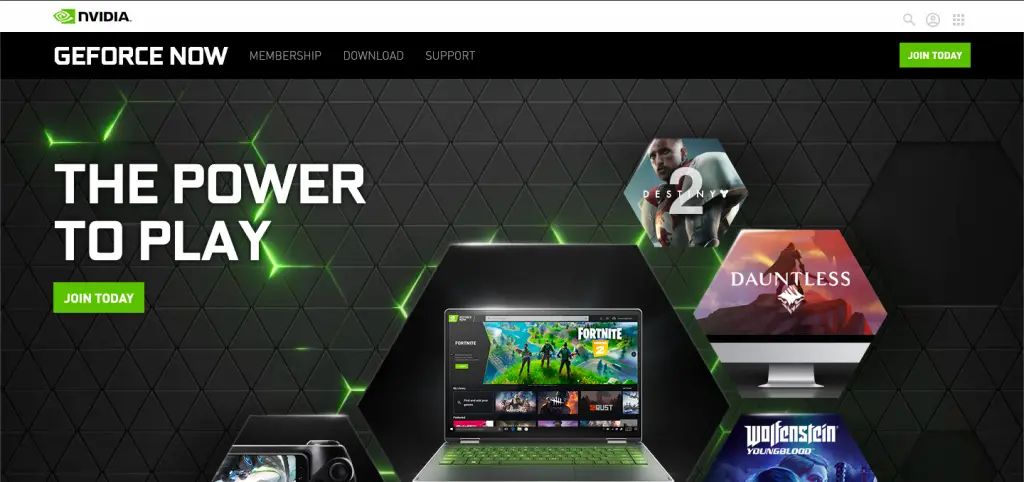The image appears to be a screenshot from the NVIDIA website, specifically promoting their GeForce Now service. Prominently displayed in the center is a sleek laptop, showcasing its integration with NVIDIA's cloud gaming technology. To the right of the laptop are three captivating screen captures from different video games, highlighting the diversity and quality of games available on the platform.

At the top left corner of the image, bold text guides the viewer with labels: "NVIDIA GeForce Now," "Membership," "Download and Support," "Join Today," "The Power to Play," and "Join Today." These headings likely direct users to various sections of the NVIDIA GeForce Now service, emphasizing the ease of accessing and joining the platform.

The photograph has a distinctive afterglow effect in the background, characterized by a neon bright green hue reminiscent of the Xbox logo, which further enhances the vibrant and modern aesthetic typical of a gaming provider's website. The overall design and color scheme align seamlessly with the dynamic and immersive experience associated with high-end gaming.